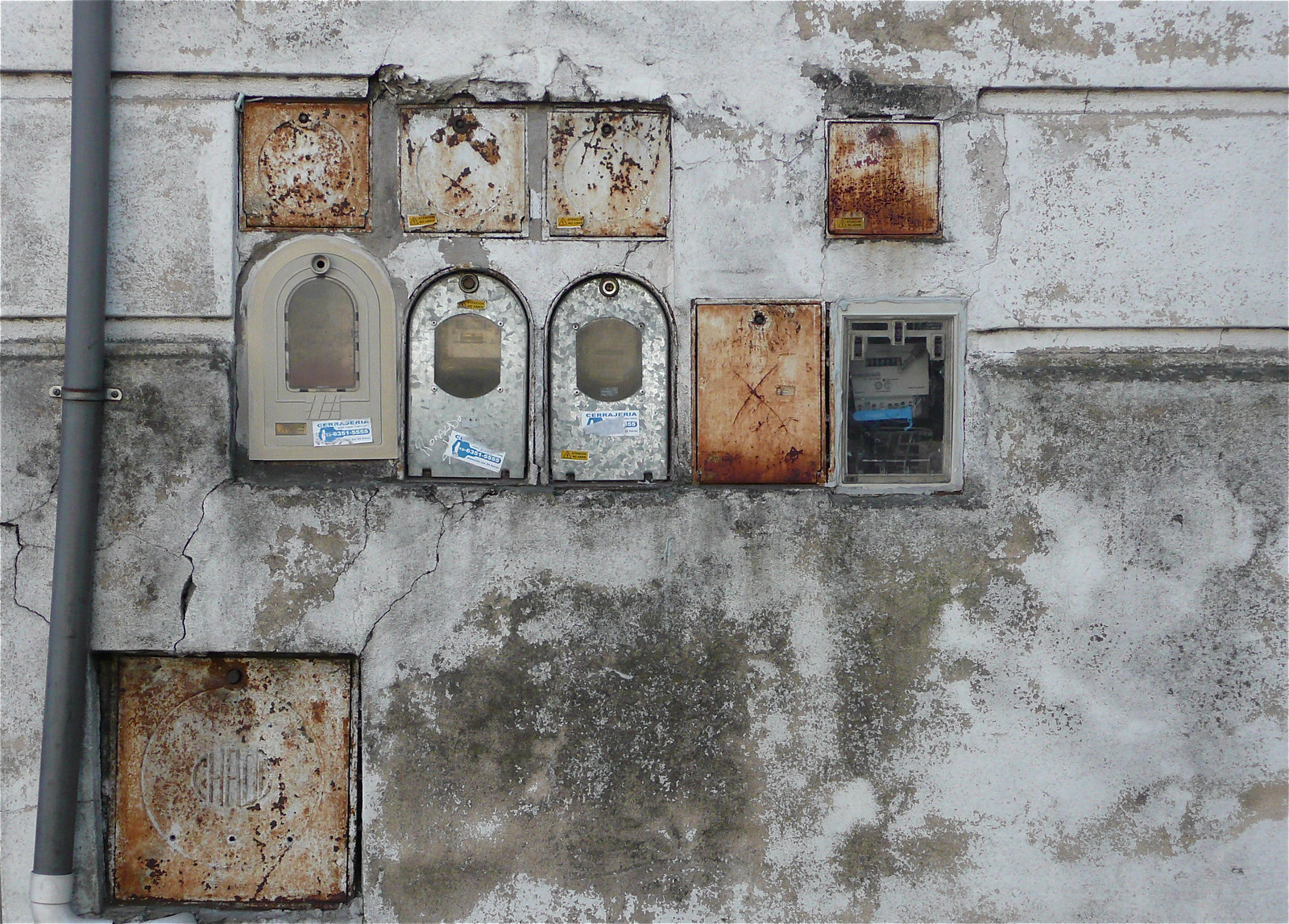This detailed photograph captures a weathered, stuccoed exterior wall of a building, characterized by mottled white, gray, and light brown hues with numerous cracks and stains from wear and exposure. Prominently featured in the lower left corner is a heavily rusted, square metal box with patches of brown and light gray. Adjacent to it on the left side, a solid gray drain pipe extends vertically from the bottom to the top of the image. 

The focal point of the wall is an indentation housing several objects. The lower section of this cutout contains an array of mailboxes with key locks, with above them, a series of four square windows in the top row, three door-like shapes on the left, and two additional square openings on the right. Some of these boxes are marked with stickers, and at least one includes a transparent window, possibly indicating an electrical meter inside. The entire wall exudes a sense of age and character, with its crusty texture and the contrast between rusted metal components and stuccoed concrete. The photograph appears to be taken in the daytime, with no visible elements other than the meticulously detailed, weather-beaten wall.